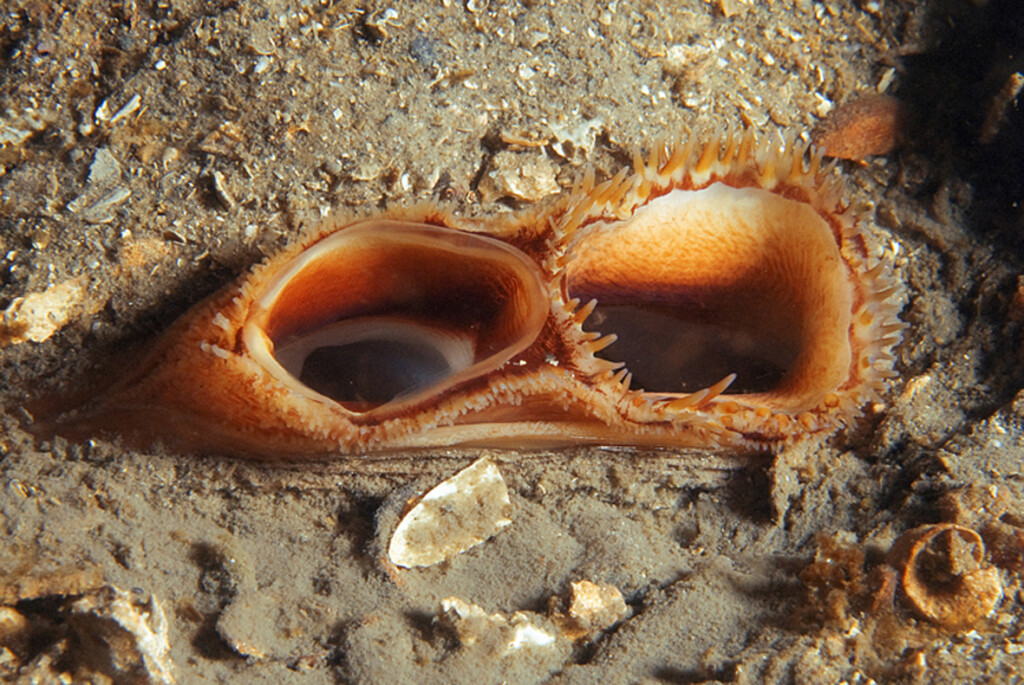This is a detailed photograph of a sandy ocean floor, approximately six inches wide and four inches high, viewed from above. The sand is a grayish-brown tone, scattered with small pebbles and bits of shells and fossils that display orange and cream-colored hues. In the upper right-hand corner, a dark, blacked-out area suggests either a shadow or a hole in the ground. At the center of the image lies a fascinating marine creature partially buried in the sand. It features two prominent holes, each about an inch wide, set against an orange-colored, coral-like structure with transparent cream-toned outlines. Thin, elongated spindles, which may resemble teeth or sensory filaments, radiate around each hole, leading inward to a smaller black hole circled by white. The overall size of this sea creature is about two to three inches wide, evoking imagery of an anemone or a bivalve, potentially functioning as a filter feeder, with its two mouths ready to capture unsuspecting prey.